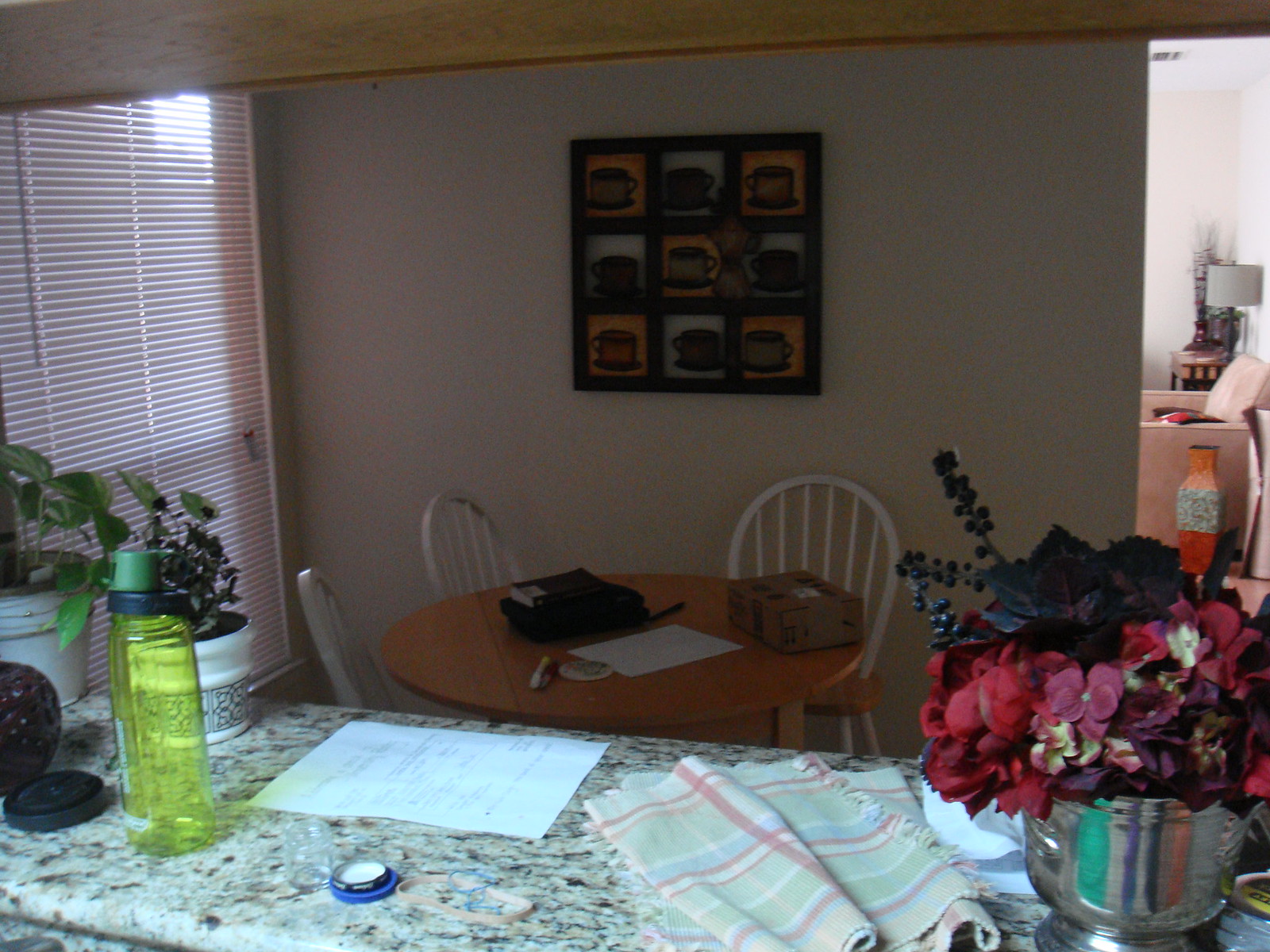A detailed and descriptive caption for the image:

The image showcases a stylish interior setup dominated by a black frame that intricately sections a photo into nine smaller, compartmentalized images. Each section features a coffee mug placed on a saucer against alternating backgrounds of yellow, orange, and blue, creating a vibrant mosaic effect. The backdrop is a pristine white wall, which contrasts with the light brown table below it. White chairs with brown seats are placed around the table, adding to the cozy atmosphere. On the right side of the table, there's a brown cardboard package. The table is adorned with scattered sheets of paper, several pens, and a sleek black book situated in the middle. In the foreground, a marble countertop holds a sheet of paper and an empty lime green water bottle. To the right of this countertop, a silver vase filled with red artificial flowers adds a touch of elegance to the scene.